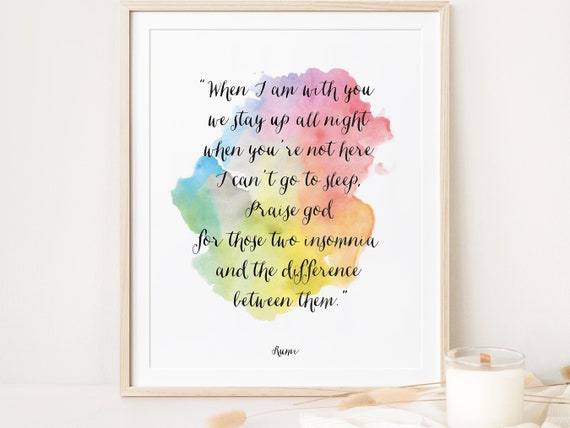The image depicts a framed saying against a light white-grey background, featuring a vibrant watercolor burst comprising reds, turquoise, pink, purple, green, blue, yellow, and orange hues. The frame, made of light tan wood, encloses the following message in black cursive lettering: "When I am with you, we stay up all night. When you're not here, I can't go to sleep. Praise God for those two, insomnia and the difference between them." Below the text, there is a signature that starts with an "L" but is too small to decipher. The artwork appears to be placed on a surface, possibly a bedside table or kitchen countertop, with a white candle and a glass of milk positioned in front of it.